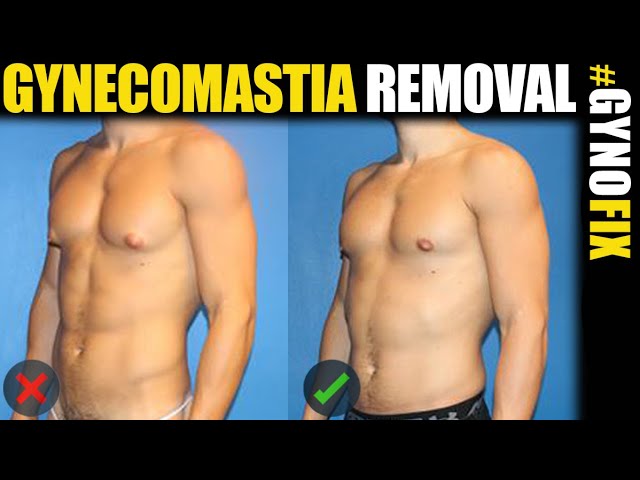The advertisement, set against a flat black background, promotes a plastic surgery procedure for gynecomastia removal. At the top of the image, "Gynecomastia" is prominently displayed in yellow font, while "Removal" is written in white. On the left side of the poster, a side-by-side before-and-after comparison showcases the transformation achieved through the procedure. The "before" image depicts a man with signs of the condition, such as a protuberance around the chest area. This image is marked with a red X in a black circle, emphasizing the undesirable state. In contrast, the "after" image on the right demonstrates a more toned and aesthetically pleasing chest, highlighted with a green check mark. The bottom right corner bears these X and check mark symbols, reinforcing the visual improvement. Additionally, running vertically along the right side of the advertisement is the hashtag "#gynofix," branding the procedure as a reliable solution for correcting gynecomastia. The entirety of the side-by-side images is set against a blue rectangle, providing a contrasting backdrop to the predominantly black layout.